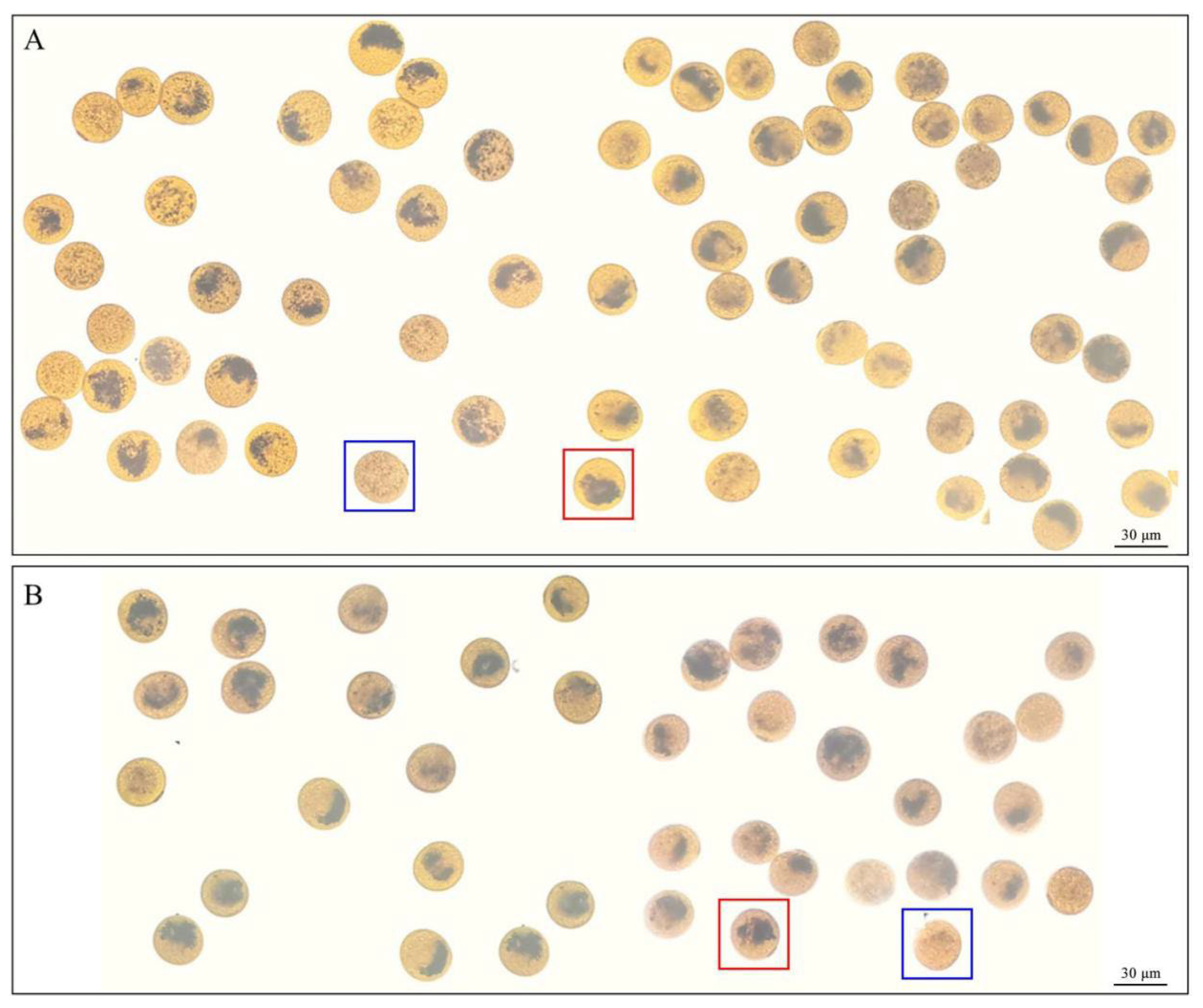The image is a detailed scientific comparison slide depicting two rectangular charts labeled A and B. Each chart is set against a white background and primarily features numerous small yellow circular objects, reminiscent of eggs or microscopic particles, some with dark masses inside. In the upper left corner of chart A is the label "A," and two specific circles are highlighted—one with a blue square indicating an empty circle, and one with a red square containing a black mass. Chart B, beneath chart A, displays similar characteristics with its own label "B" in the upper left corner. The circles in chart B are slightly less vibrant compared to chart A. Like chart A, chart B has two highlighted circles; in this instance, the red square is on the left and the blue square is on the right. Both charts feature a scale marker in the bottom right corner, labeled "30µm," suggesting a microscopic scale. The overall style of the image suggests a photorealistic, scientific approach, likely taken from a microscope slide, for comparative analysis.